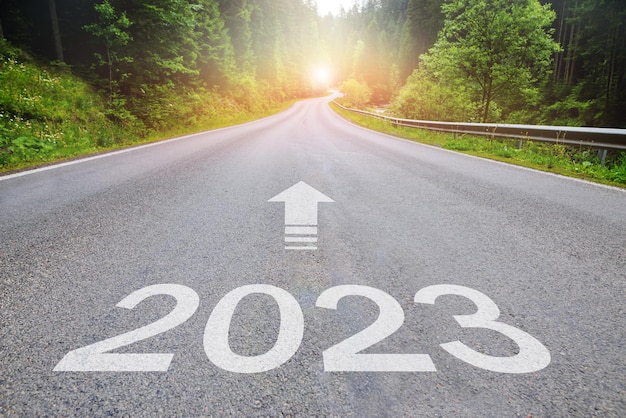In this image, we see a low-angle shot from a camera positioned just above the gray asphalt of a road, capturing a close-up view of white-painted numbers "2023" along with an arrow pointing forward. This scene is likely a metaphor for journeying through the year 2023 or anticipating its arrival. The road extends into the distance, flanked on both sides by a dense, heavily wooded area populated with a variety of trees, shrubs, and other vegetation, suggesting a forested or rural setting. There are both deciduous and evergreen trees visible, indicating a season when the flora is lush and green, likely summertime. To the right, a metal guardrail is present, ensuring cars stay on the road and don't veer off into the underbrush. In the background, at approximately street level, there is a bright glare, possibly from a reflection or an artificial light source. The image is serene yet evokes a sense of forward movement and anticipation as one looks down the road toward the metaphorical journey of 2023.